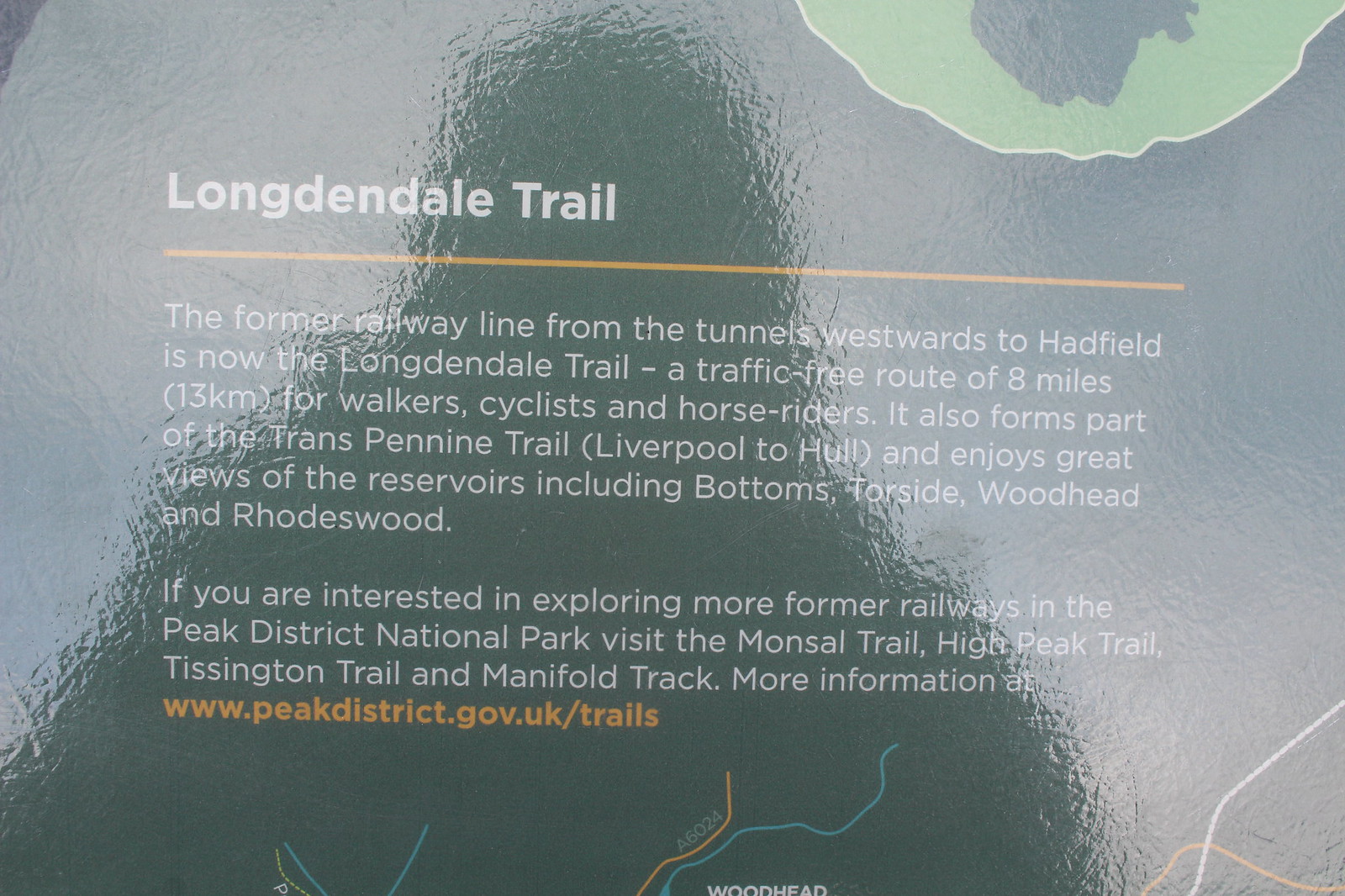The image captures a shiny, possibly metal or plastic plaque situated outdoors, reflecting the silhouette of the person taking the photo. The plaque has a greenish-gray background with white text. It prominently features the title "Longdendale Trail" in bold white letters, located at the top left corner, followed by an orange line beneath it. The text reads: "The former railway line from the tunnels westwards to Hadfield is now the Longdendale Trail, a traffic-free route of eight miles for walkers, cyclists, and horse riders. It also forms part of the Trans-Pennine Trail, Liverpool to Hull, and offers great views of reservoirs including Bottoms, Torside, Woodhead, and Rhodeswood." Below this, there is more information and a partial view of a local map displaying various trails in different colors. The plaque also mentions exploring additional trails like the Monsal Trail, High Peak Trail, or Tissington Trail, and provides a contact link at peakdistrict.gov.uk/trails.